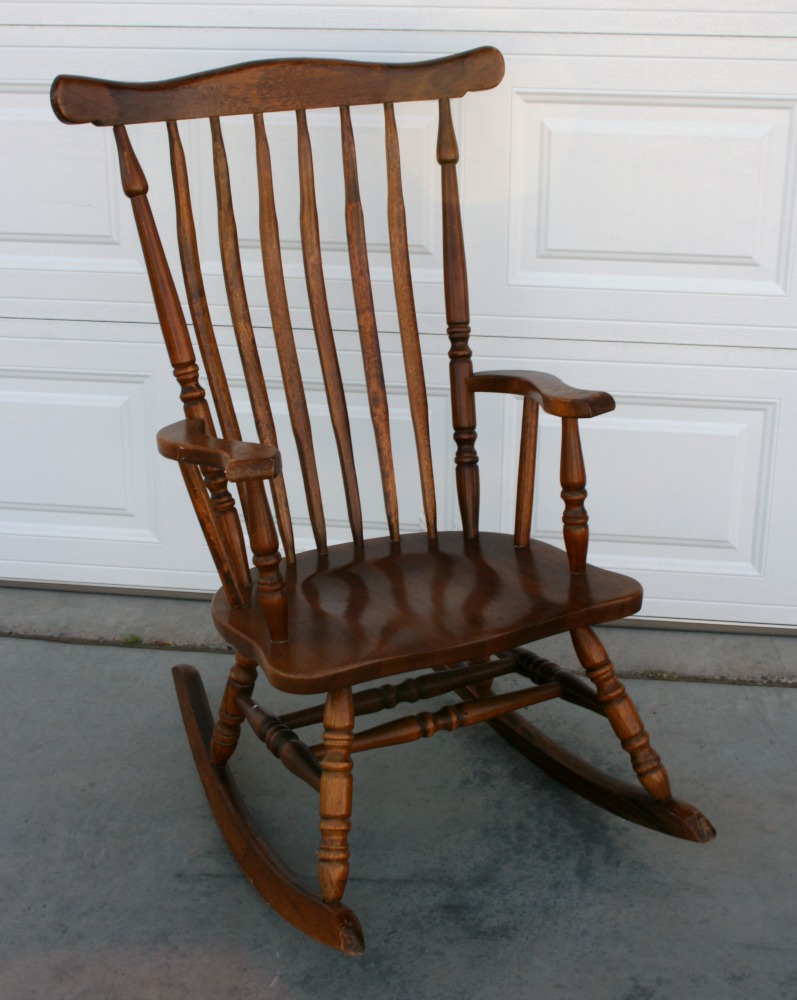The image features a traditional wooden rocking chair set on a gray concrete surface, likely outdoors. Behind the chair is a white garage door with segmented, rectangular panels. The rocking chair itself is crafted from wood with a dark, glossy finish, possibly coated with shellac. It has seven vertical slats on the backrest, and flat armrests on either side. The seat is a very dark brown, contrasting slightly with the lighter brown hue of the rest of the chair. The chair's base includes four horizontal support bars, two extending directly below the seat and two crossing beneath to enhance stability. The curved wooden pieces attached to the bottom of the legs enable the chair to rock back and forth. The scene appears to be illuminated by natural daylight.